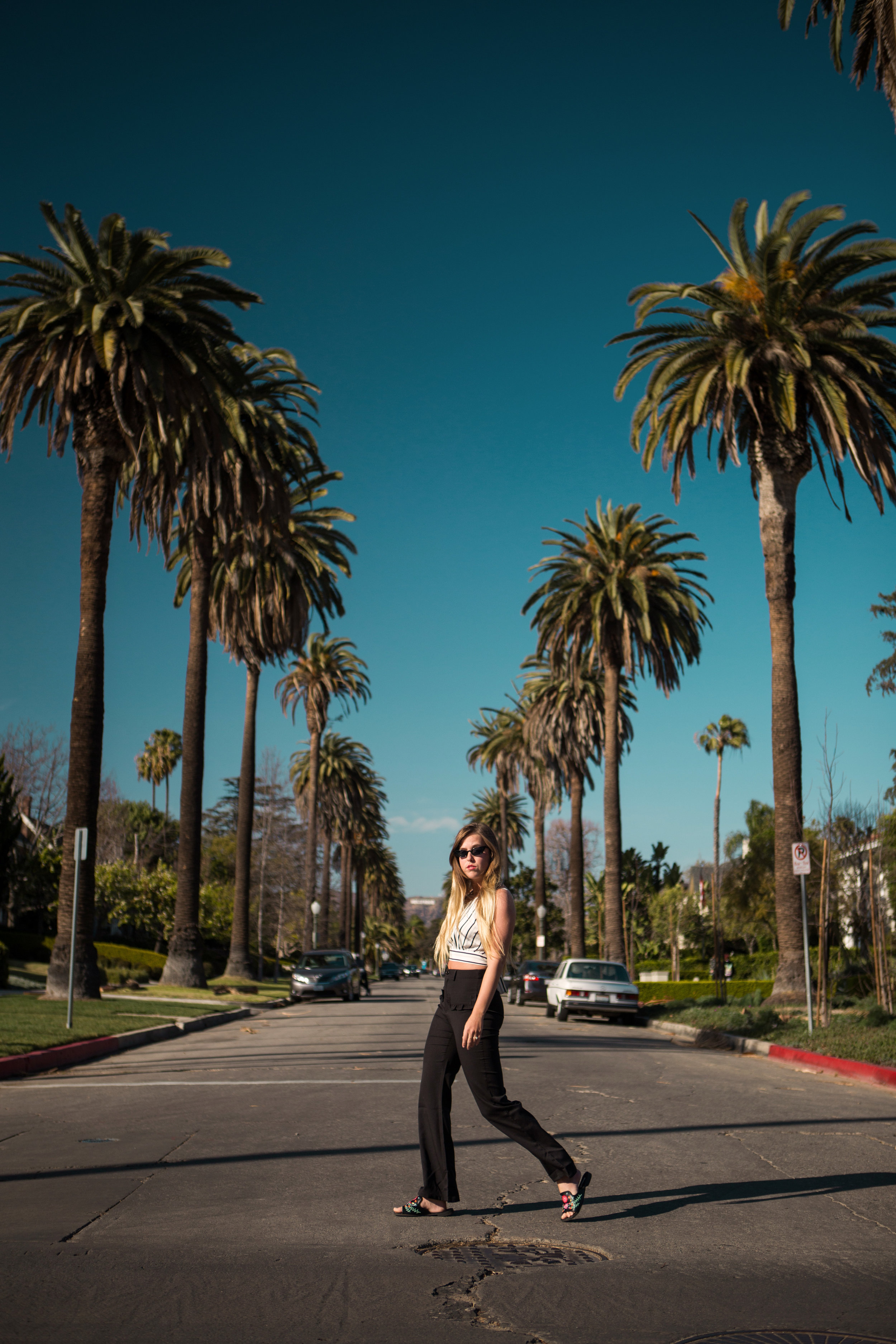In this detailed photograph, a young woman with long blonde hair is crossing a residential street lined with tall, manicured palm trees. The street, which has some cracks in the pavement, is dark gray and extends into a clear sky that transitions from a rich, darker blue at the top to a serene, Tiffany blue near the horizon. The woman is positioned centrally in the image, moving from the right towards the left, with her gaze directed towards the camera, a hint of red lipstick visible on her fair-skinned face. She is dressed in a stylish ensemble comprising a white sleeveless top, exposing her shoulders and midriff, and black, flowy pants. Her feet are adorned with black slide sandals decorated with red and green designs. Her left arm hangs naturally by her side, while her right arm is hidden from view. Black sunglasses shield her eyes, adding a touch of chic mystery. The street behind her features parked cars, including a white car on the right side, adjacent to a red-painted curb, enhancing the organized, suburban feel of the location. The overall ambiance suggests a warm, sunlit climate, likely a place reminiscent of Florida or Las Vegas.